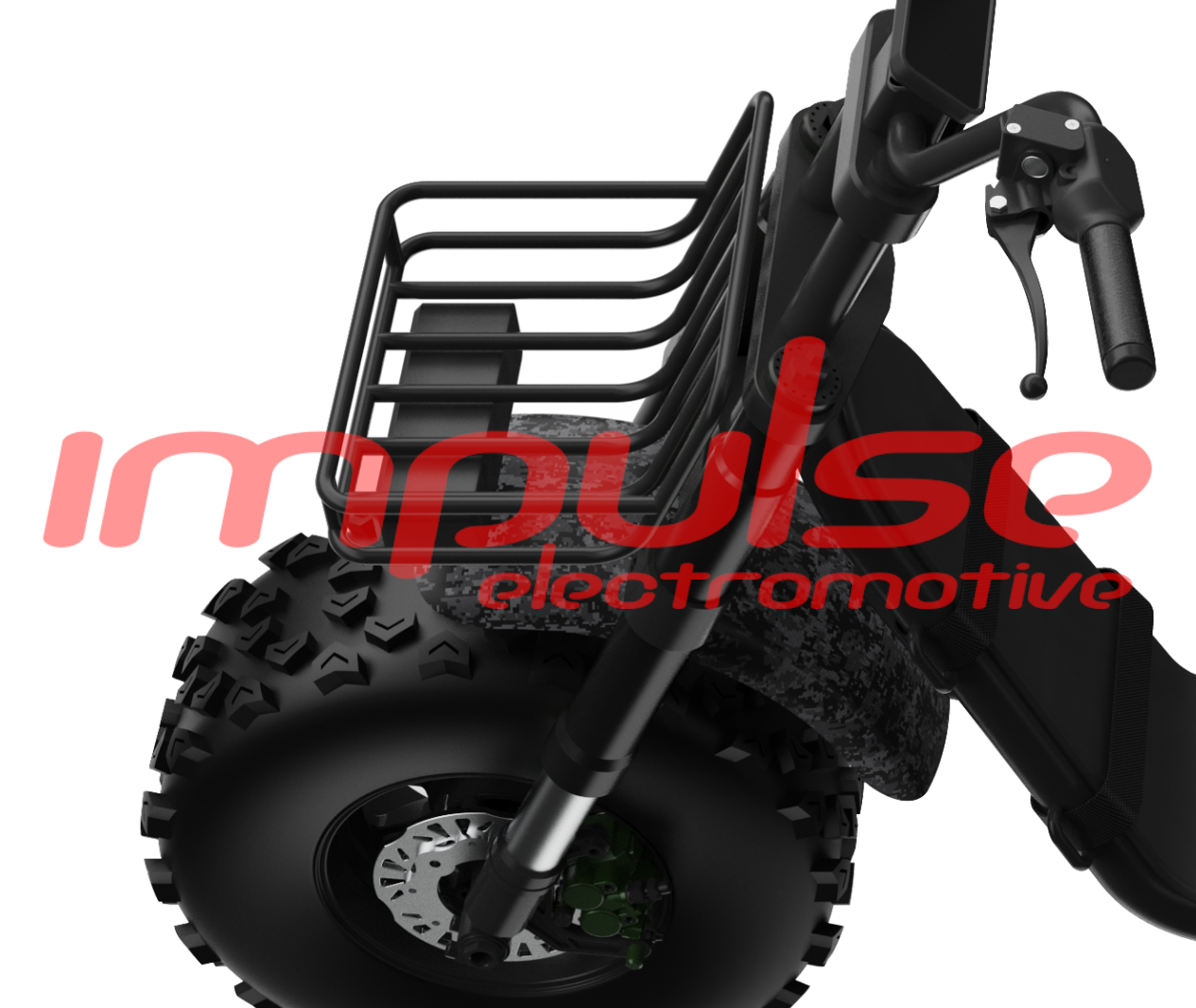The image showcases the front portion of a sleek electric scooter or motorcycle against a white background. The focus is on the black, matte-finished handlebar area, leading down to a robust fork and a notably thick and rugged tire, approximately 20 inches in diameter and 6 inches wide, with distinctive demarcations suggesting it's designed for off-roading. Attached above the tire is a metal basket or crate, suitable for carrying small items, indicating practicality for commuting or casual use. A brake handle is visible, adding to the detailed view of the scooter's front assembly. The brand name "Impulse Electromotive" is prominently displayed in red font across the middle of the image, likely suggesting a watermark. Additionally, the plate above the tire bears a faint dark camo pattern, adding a subtle design element to the overall aesthetic. The high-quality construction and design elements suggest that this is a premium electric scooter, ideal for daily transit.